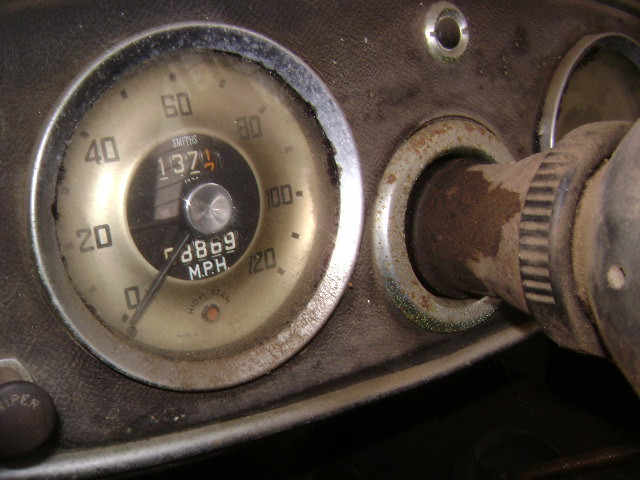The image depicts the interior of a vintage car, estimated to be between 80 to 100 years old. The focal point is an old-fashioned, heavily rusted speedometer gauge that measures speed from 0 to 120 miles per hour. The gauge has a gray background with large black numerals, and the odometer displays a mileage of 68,869 miles. To the right of the speedometer, there is a very rusty and dusty steering wheel. On the left side of the speedometer, a button is visible with partially legible letters "I-P-E-R." Above the steering wheel, and to the right of the speedometer, there's another button, although the specifics are unclear. The overall scene conveys a sense of antiquity and decay, capturing the historical essence of the vehicle.